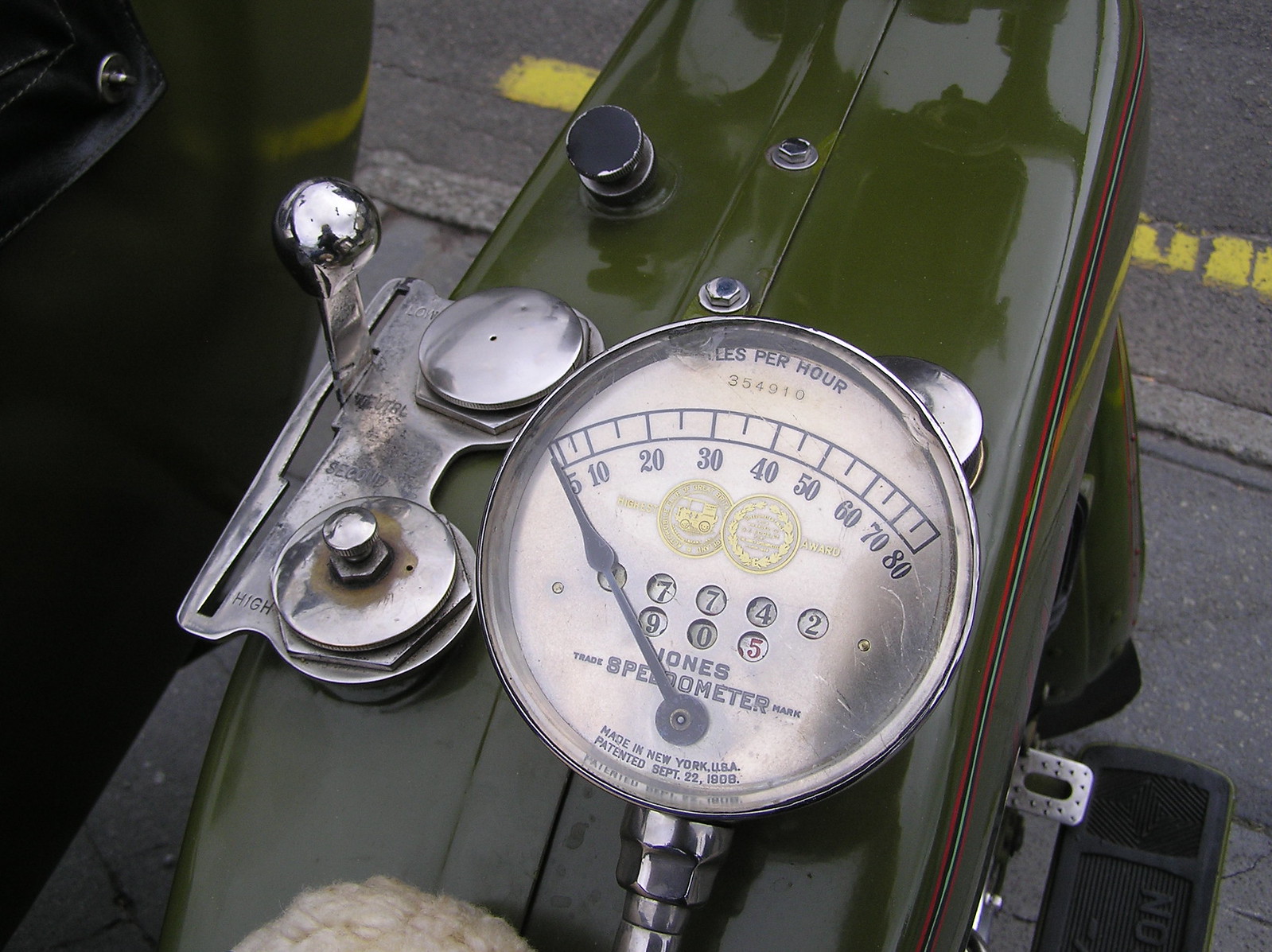This photo features a vintage bike, showcasing a number of components from an earlier era. The bike's frame is a lustrous olive army green, suggesting it has either been freshly painted or meticulously maintained over the years. To the left, the gear system is visible, allowing shifts between neutral, second, and high gears. This component is chrome-plated, though some wear and slight distortion are evident, highlighting its age and usage.

Centrally located in the image is a classic speedometer. The gauge displays speeds in miles per hour, with numerical markings ranging from 5 to 80. At the top of the speedometer, the text "miles per hour" is inscribed, followed by the numbers "354910" just below it. Underneath these numbers, the reading "17742" appears, indicating the total mileage, with "905" positioned directly below.

The face of the speedometer is branded with "Jones Speedometer," noted as a trademarked product made in New York, USA. Additionally, the speedometer's patent date is marked as September 22, 1908, providing historical context to the instrument’s manufacture. This vintage detail contributes to the overall nostalgia and charm of the bike.